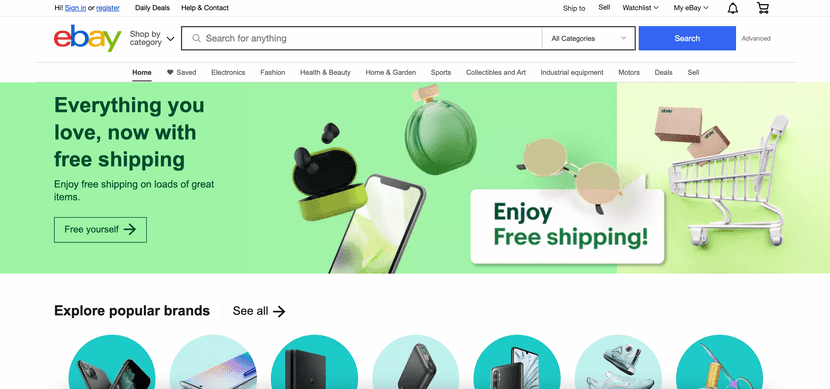This is a cleaned-up and detailed caption for the described image:

---

This is a screenshot of the front page of eBay. In the upper left-hand corner, the site prompts users with "Hi, Sign In or Register," with both "Sign In" and "Register" presented as blue clickable links. Next to these are links for "Daily Deals," "Help & Contact." On the right-hand side, options for "Ship To," "Sell," "Watchlist," "My eBay," a notifications icon, and a shopping cart icon are displayed. 

Centered on the page is the iconic eBay logo, with the 'e' in red, 'b' in blue, 'a' in yellow, and 'y' in green. Below this, a search bar spans the width of the page, containing the text, "Shop by category, search for anything," along with a dropdown menu labeled "All Categories," a blue search button, and an "Advanced" link.

The navigation bar beneath the search bar features categories including: "Home," "Saved," "Electronics," "Fashion," "Health & Beauty," "Home & Garden," "Sports," "Collectibles & Art," "Industrial Equipment," "Motors," "Deals," and "Sell," with "Home" being highlighted.

A green border prominently features the message, "Everything you love now with free shipping. Enjoy free shipping on loads of great items for yourself." This is accompanied by an illustration of a shopping cart filled with various items like boxes, sunglasses, fragrances, a cell phone, and earbuds.

Following this section, in bold black text, it reads "Explore popular brands," next to a "See All" link. Towards the bottom of the screenshot, partial images and seven blue-colored circles containing various items are visible, though they are cut off at the bottom of the image.